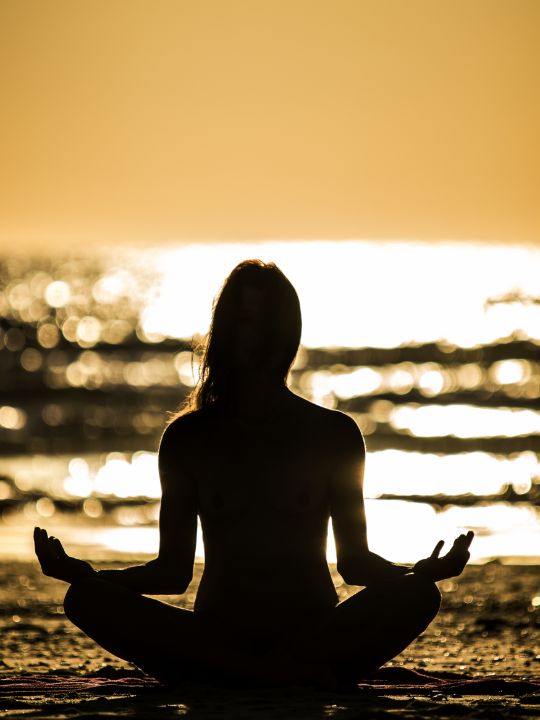In this evocative photograph, a woman is silhouetted against the backdrop of a serene beach at sunset. Seated cross-legged directly on the damp, shimmery sand, she faces the ocean, her posture erect. Her arms rest on her knees, with her palms open upwards in a classic yoga pose, exuding tranquility and mindfulness. The setting sun casts a warm glow, tinting the image in hues of black, white, and mustard yellow, creating a striking contrast against her shadowed form. The background, though blurred, suggests a glimmering ocean and a golden, orange-tinged sky, adding to the tranquil atmosphere of the scene. Her long hair, swept over one shoulder, and her fit physique further emphasize her peaceful engagement with the beautiful, almost meditative setting.